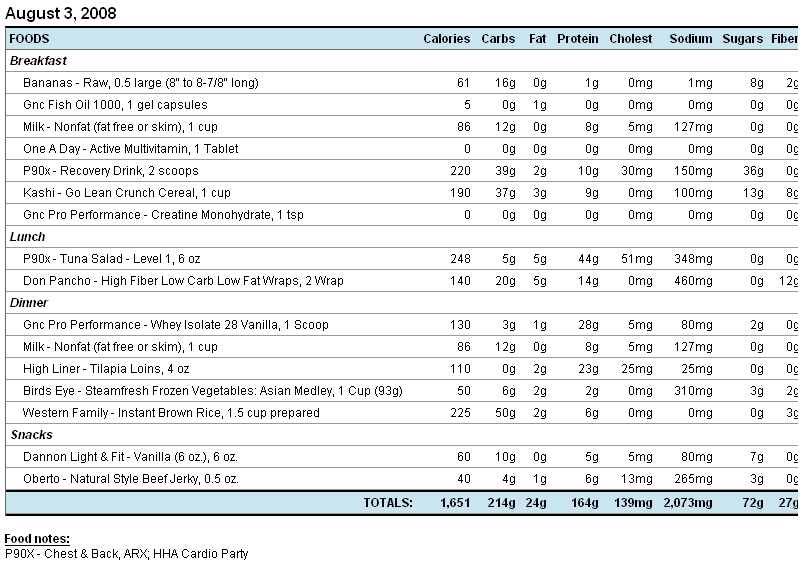This image captures a detailed nutritional chart dated August 3rd, 2008. The chart meticulously logs the foods consumed throughout the day, categorized into breakfast, lunch, dinner, and snacks, with each food item's nutritional breakdown listed. At the top of the chart, headings in black print on a light blue background indicate key nutritional metrics: calories, carbs, fat, protein, cholesterol, sodium, sugars, and fiber. 

For breakfast, the chart includes entries like "bananas, raw, 0.5 large (8 to 8 7/8 inches)" with detailed nutritional values, alongside items like "GNC fish oil (1,000 mg, 1 gel capsule)", "milk, nonfat (1 cup)", "1 a day active multivitamin (1 tablet)", "P90X recovery drink (2 scoops)", "cashew go lean crunch cereal (1 cup)", and "GNC pro performance creatine monohydrate (1 teaspoon)". 

Lunch includes "P90X tuna salad (level 1, 6 ounce)" and "Don Pancho, high fiber, low carb, low fat wraps (2 wraps)". Dinner lists items such as "GNC pro performance whey isolate (28 vanilla, 1 scoop)", "milk", "high liner tilapia loins", "Bird's Eye frozen vegetables, steamed", and "Western Family brown rice". 

Snacks feature "Dannon Light & Fit vanilla yogurt" and "Oberto natural style beef jerky". The chart also tallies total nutritional values at the bottom and includes a 'food notes' section in the lower left corner. This comprehensive approach helps in tracking overall daily calorie and carbohydrate intake, among other nutritional data, highlighting the user's aim for detailed dietary monitoring.